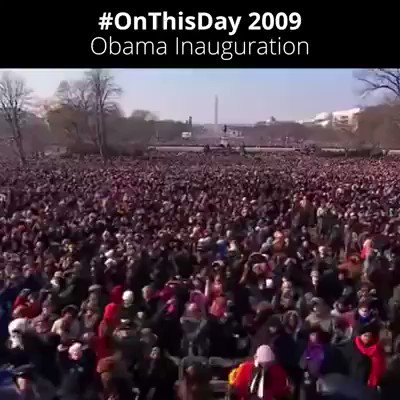A large crowd gathers in front of the Washington Monument, celebrating the 2009 Obama inauguration. At the very top of the image, white text overlaid on a black rectangular background reads "#OnThisDay 2009 Obama inauguration". Bare trees, signaling fall or winter, frame the scene, their leafless branches contrasting with a cloudless sky. The vast assembly of people, dressed in winter attire with colors including red, black, purple, and white, stretches into the distance. Despite some blurriness, the energy and historical significance of the moment are palpable.